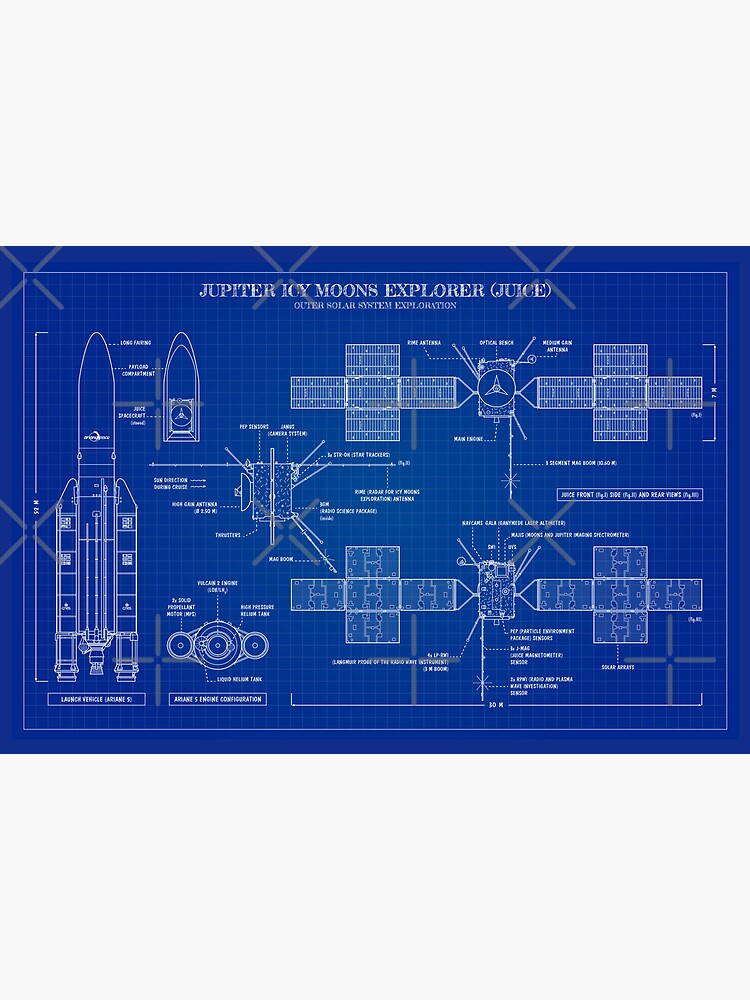The image depicts detailed blueprints of the "Jupiter Icy Moons Explorer" (JUICE) mission, intended for outer solar system exploration. The title, "Jupiter Icy Moons Explorer (JUICE)," is prominently displayed in larger, white font in the center of the blueprint, with the subtitle "Outer Solar System Exploration" in brackets below. The background is a deep blue, and all text and drawings are rendered in white, although some smaller text is difficult to read due to its size.

On the far left, a detailed drawing of a rocket is featured, consisting of a central main rocket flanked by two side boosters. Although there is text beneath the rocket, it is too small to be legible. The blueprint zooms in on key sections of the rocket, showing intricate details at the tip and the main engine area below.

In the center of the blueprint, there is a detailed examination of what appears to be a tubular section with several solar panels depicted, arranged around a central circular component, resembling a switch point with triangular blades.

To the right, additional drawings show more components, including what looks like solar panels and a box-like structure. At the lower-left section of the blueprint, three interconnected circles are depicted, one larger central circle flanked by two smaller circles connected by lines, possibly representing part of the spacecraft's inner wiring or structural components.

Overall, the blueprint is a detailed and intricate guide for constructing a spacecraft designed to explore Jupiter's icy moons, with an emphasis on various components and their configurations.